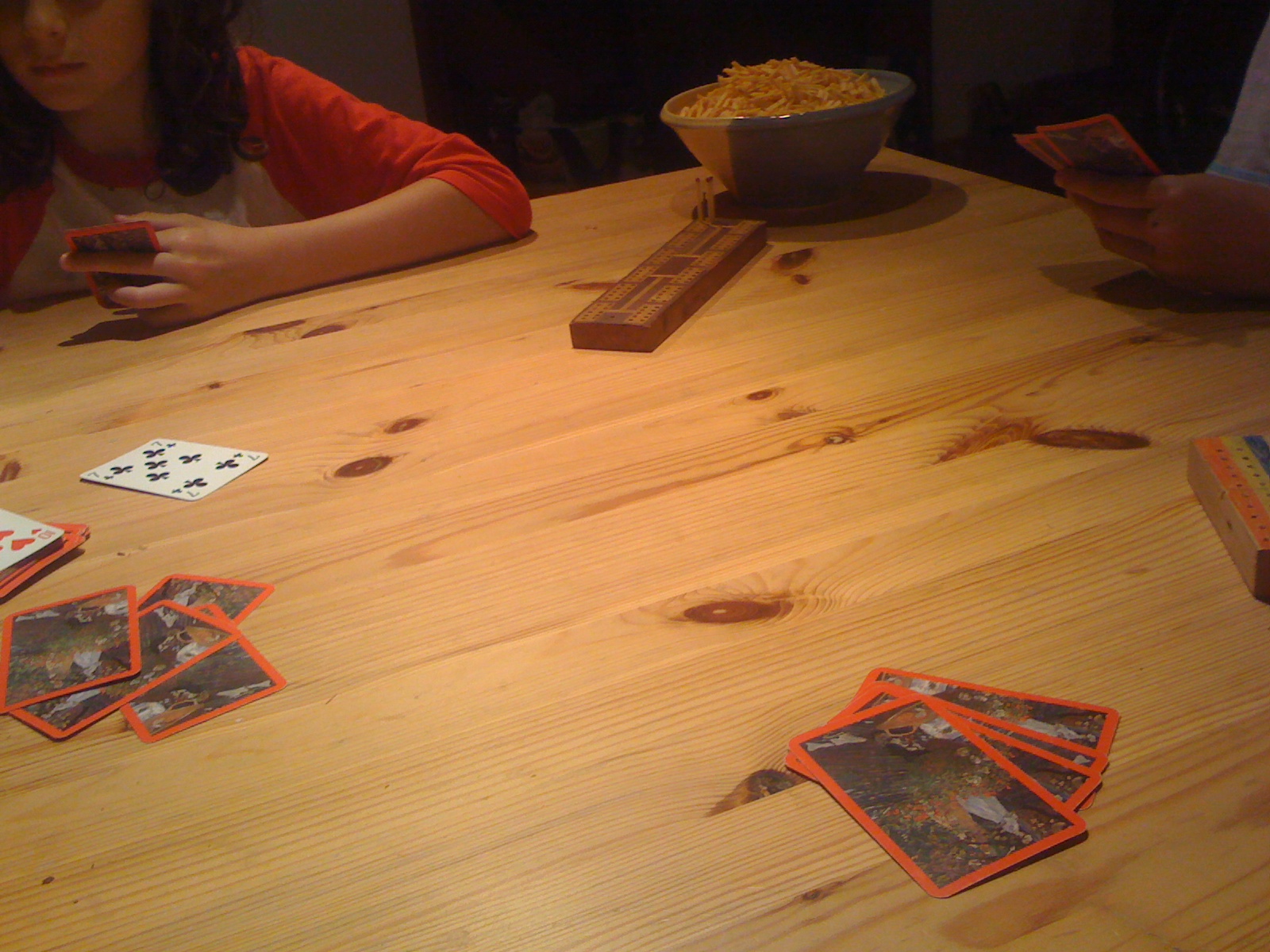In this detailed image, we are peering downward at a smooth, wooden table from an approximate 35-degree angle. The table features a variety of elements, predominantly playing cards. In the bottom right corner of the image, four cards are laid face down, each adorned with an orange border and faint scenery that resembles leaves.

Towards the rear of the table, a person is seated, though their identity remains partly obscured as the top half of their face is cut off from view, leaving only their nose and mouth visible. They maintain a neutral expression. The individual wears a shirt with orange sleeves reaching up to the elbows and a white torso. Their arm is resting on the table, holding one of the face-down cards between their index and middle fingers.

Closer to us, on the left side of the image, there are more playing cards. A Seven of Clubs and a Ten of Hearts are face up, with the Ten of Hearts positioned atop a stack of face-down cards. 

In the image's upper middle section, slightly off to the right, a large, bluish-gray bowl filled with chips is visible. Below the bowl lies a rectangular wooden object peppered with holes, from which two matches protrude upwards. 

Finally, at the very top right of the image, another hand is visible, clutching two or three card backs, adding to the card game ambiance captured in the scene.